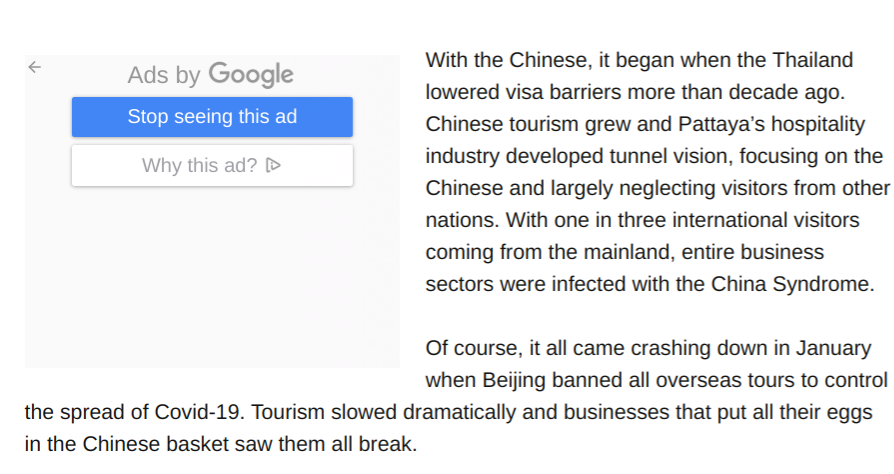The image is a snippet of a webpage with a predominantly white background. On the left side, there is a very light gray square, featuring various text and interactive elements associated with Google Ads. At the top of the gray square, in lighter gray text, it says "Ads by Google," with the Google logo also rendered in gray rather than its usual colorful form. Below this, there is a blue rectangle with white font that states, "Stop seeing this ad." Underneath this blue rectangle, there's a white rectangle with gray font reading, "Why this ad?" followed by a right-pointing triangle, indicating that clicking this would likely take the user to another webpage with more information about the ad.

To the right of this ad section, the snippet reveals part of an article. This article is presented in gray font and includes a full paragraph and part of another. The text begins with, "With the Chinese, it began when Thailand lowered visa barriers more than a decade ago," and continues to describe how Chinese tourism grew, leading to a focus on Chinese visitors in Pattaya's hospitality industry, while other nationalities were largely neglected. The visible part of the article concludes mid-sentence, with additional blank space beneath it. The webpage's source and further content are not visible in this snippet.